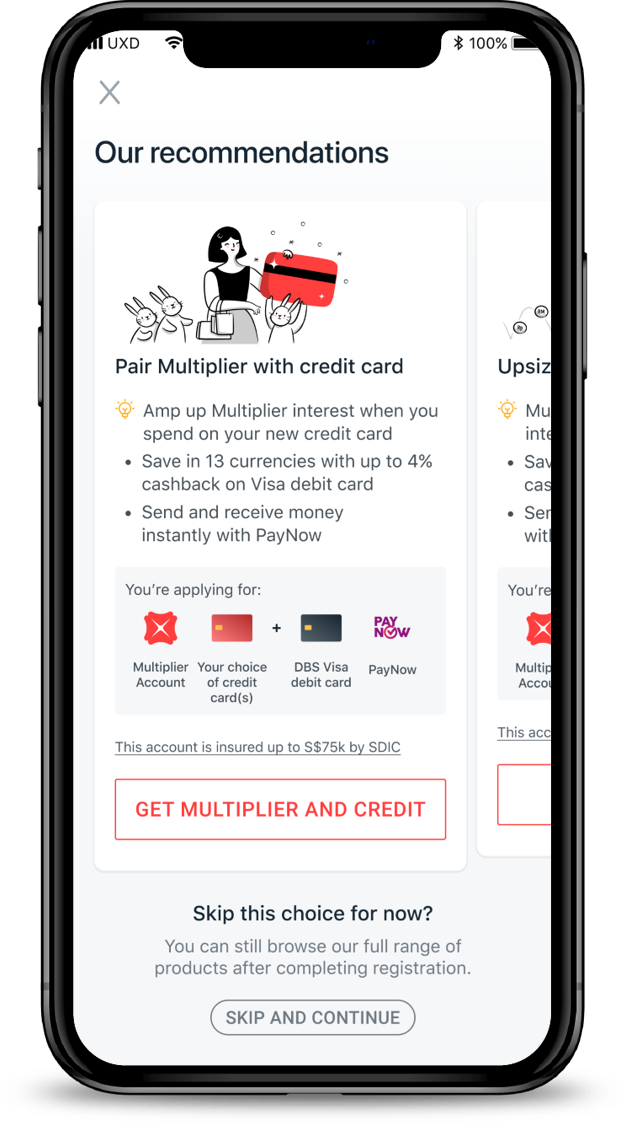This image depicts a smartphone screen showcasing a banking application interface. In the top-left corner, the status bar displays full signal strength, a Wi-Fi icon, and on the top-right, there is a Bluetooth icon alongside a 100% battery indicator. The main section of the screen features a promotional message recommending the "Multiplier" account and associated credit card. 

The message encourages users to pair the Multiplier account with a credit card to enhance interest earnings, save in 13 different currencies, and earn up to 4% cash back with a Visa debit card. The screen also mentions the ability to send and receive money instantly with the "Pay Now" feature. The visual design includes whimsical illustrations of rabbits surrounding a woman shopping, with one rabbit holding a large credit card, visually reinforcing the promotional content.

There is a button to proceed with applying for the Multiplier account and credit card, and a "Skip This Choice" option that allows the user to browse other offers after completing registration. Additionally, the layout suggests the presence of more navigational options accessible by scrolling left, though these are not visible in the current frame. Overall, the scene indicates that the user is in the process of exploring or signing up for financial products via the banking app.